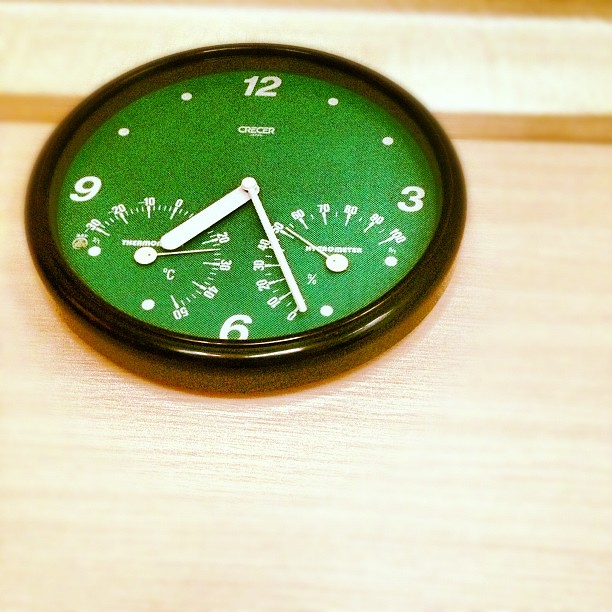The image features a glossy black-framed, round wall clock positioned against a very light horizontal wood grain background, viewed from a slightly downward angle. The clock face is a shiny, grass green color adorned with white Arabic numerals at the 12, 3, 6, and 9 positions, with the remaining hours marked by white dots. There are two white hands indicating that the short hand falls between 7 and 8, while the long hand is between 5 and 6. At the top of the clock face, a name is written in white. The bottom right of the clock includes two additional dials: one is a thermometer reading approximately 24 degrees Celsius, located between the 9 and 6 positions, and the other is a hydrometer reading 50 out of 100, situated between the 3 and 6 positions.